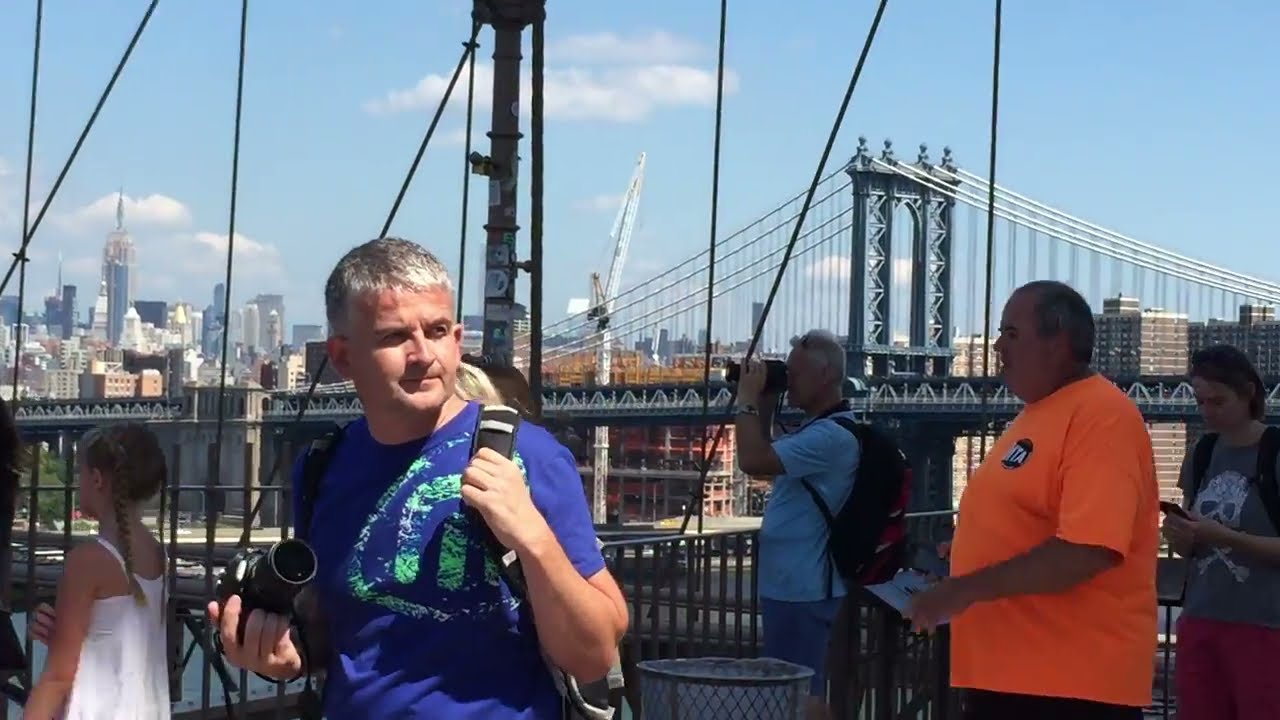The photograph captures a lively, sunlit scene on a wooden walkway portion of a suspension bridge in New York City. In the forefront on the right-hand side, a Caucasian woman with light brown hair pulled back into a ponytail strides towards the right. She sports aviator sunglasses and a black, white, and red striped tank top with geometric designs, highlighting her casual summer attire. Behind her, about four paces, another Caucasian woman, also wearing sunglasses, dons a blue ball cap with 'NYC' emblazoned on it, paired with a light gray v-neck tank top and black shorts. To her left, with her back facing the viewer, a woman with shoulder-length gray hair is seen in a straw-brimmed hat and a white, pink, and purple plaid long-sleeved button-up shirt, with a black handbag slung over her shoulder. In the center, a man rides a bicycle, a backpack slung over his shoulders, contributing to the bustling energy of the scene. The background reveals the expansive cityscape of New York City under a partly cloudy, bright blue sky. Another iconic suspension bridge towers in the distance, reinforcing the characteristic urban setting. The image vividly captures the essence of a warm summer day, with the reflection of the water visible beneath the boardwalk, indicating the bridge's elevation over the river.